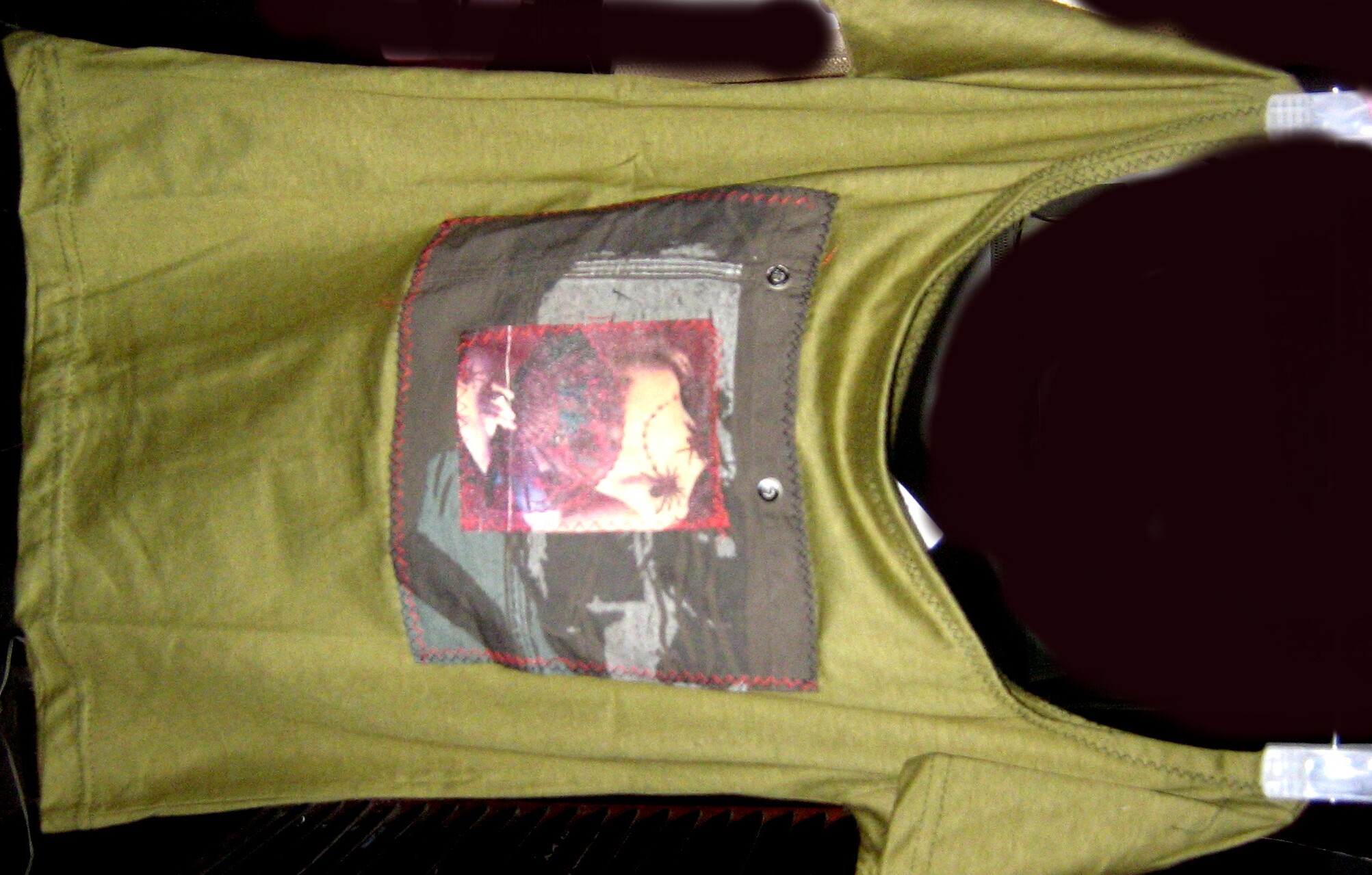This photograph features a women's shirt displayed sideways, as if hung on a coat hanger not visible in the frame. The shirt has a broad, open neckline and comes in a unique light orangey-green camouflage pattern. On the front, there's a layered design: a photograph of a woman holding a red fan, overlaid on another image that appears to be in grayscale, possibly a graphic drawing. The contrast between these images and the shirt's background, which is predominantly black—whether from shadows or the fabric itself—creates a striking visual. Notably, there are illustrations of spiders crawling on the woman in the photograph, adding a gothic, grungy aesthetic to the overall design. The shirt also features two buttonholes, though other details are difficult to discern due to the dark background.